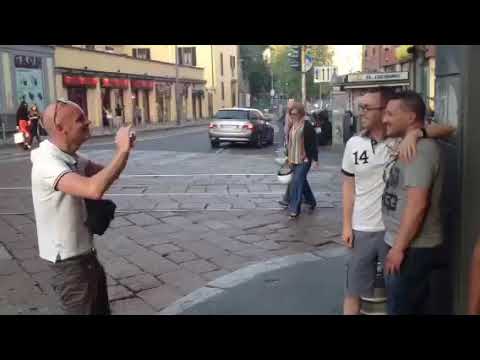In this photograph, we see a bustling, cobblestone street in what appears to be a touristy town. Centered in the image is a scene where a bald man, dressed in a white t-shirt and dark slacks, is capturing a moment with his camera. He stands poised and smiling as he takes a picture of two men posing together. One man, adorned in a white polo shirt displaying the number "14" and gray shorts, has his arm around the shoulder of the second man, who is dressed in a gray t-shirt and jeans. Both men are smiling and facing slightly away from the camera, caught in a candid side view. Surrounding this trio, the street is animated with people walking, and a car is parked nearby. The sides of the street are lined with buildings and shops, including a prominent large yellow-painted building. Street signs signal various directions, adding to the everyday yet lively atmosphere of this charming, dark-brown, rectangular-brick road.